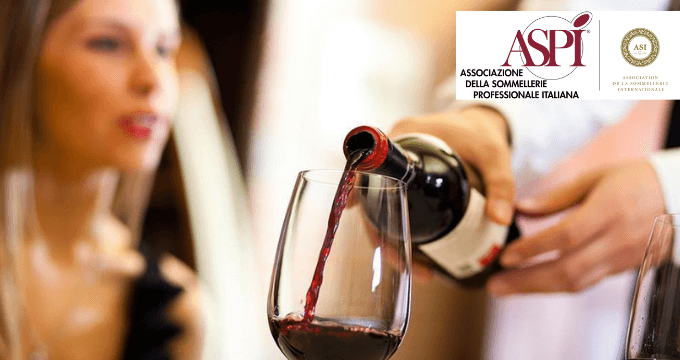In this detailed and vibrant color photograph with a landscape orientation, the primary focus is on a person pouring red wine from a black bottle into a tall, clear wine glass situated at the center of the image. The hands of the individual, who is dressed in a long-sleeved white shirt, are visible on the right-hand side, skillfully pouring the wine. The wine glass shows a modest amount of red wine, about 20% full, and the bottle, which has a white rectangular label and red foil around the opening, is positioned horizontally behind it.

To the left of the image stands a slightly out-of-focus woman dressed in a black outfit with straight, dirty blonde hair that falls to just above her breasts. She wears pink lipstick and is gazing towards the action of the wine being poured.

The upper right corner of the picture features a detailed emblematic representation. A white horizontal rectangle displays text in burgundy capital letters reading "ASPI," with a black circle behind it. Beneath this, in black text, it states "Associazione della Somamlieri Professionale Italiana." Adjacent to this, further to the right, lies another circular logo in gold with additional, smaller text that's illegible. The colors present in the photograph include olive, brown, red, purple, clear, and olive, contributing to the overall realistic and representational graphic design feel. The entire scene appears to be set within a sophisticated restaurant environment.